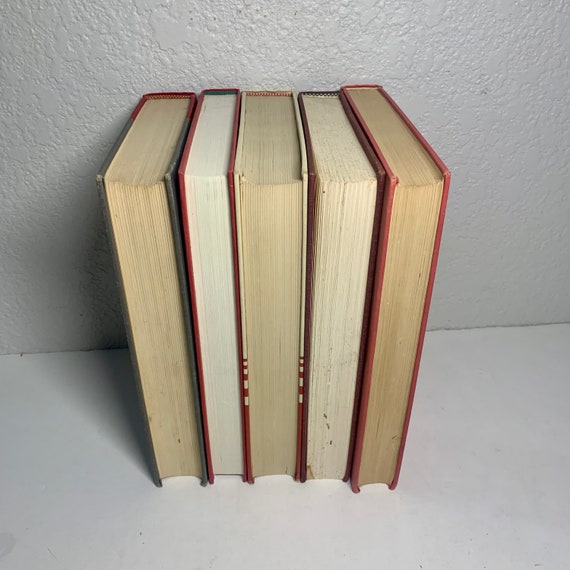The photograph features five hardcover books standing vertically on a gray stone-like surface against a worn and chipped gray wall. The spines of the books are facing the wall, exposing the pages to the viewer. From left to right, the first book has a red spine with green front and back covers; its yellowing pages suggest it's well-aged. The second book, outlined in red, has noticeably white pages. The third book, equally as thick as the first, also has yellowing pages and its cover shows a mix of yellow and red shades. The fourth book, with a brown cover, has slightly yellowed pages but not as pronounced as the previous ones. The final book has a light red cover and very dirty, dingy yellow pages. The arrangement and various colors of the books' covers, ranging from shades of red and brown to off-white, add to the visual interest of the image.